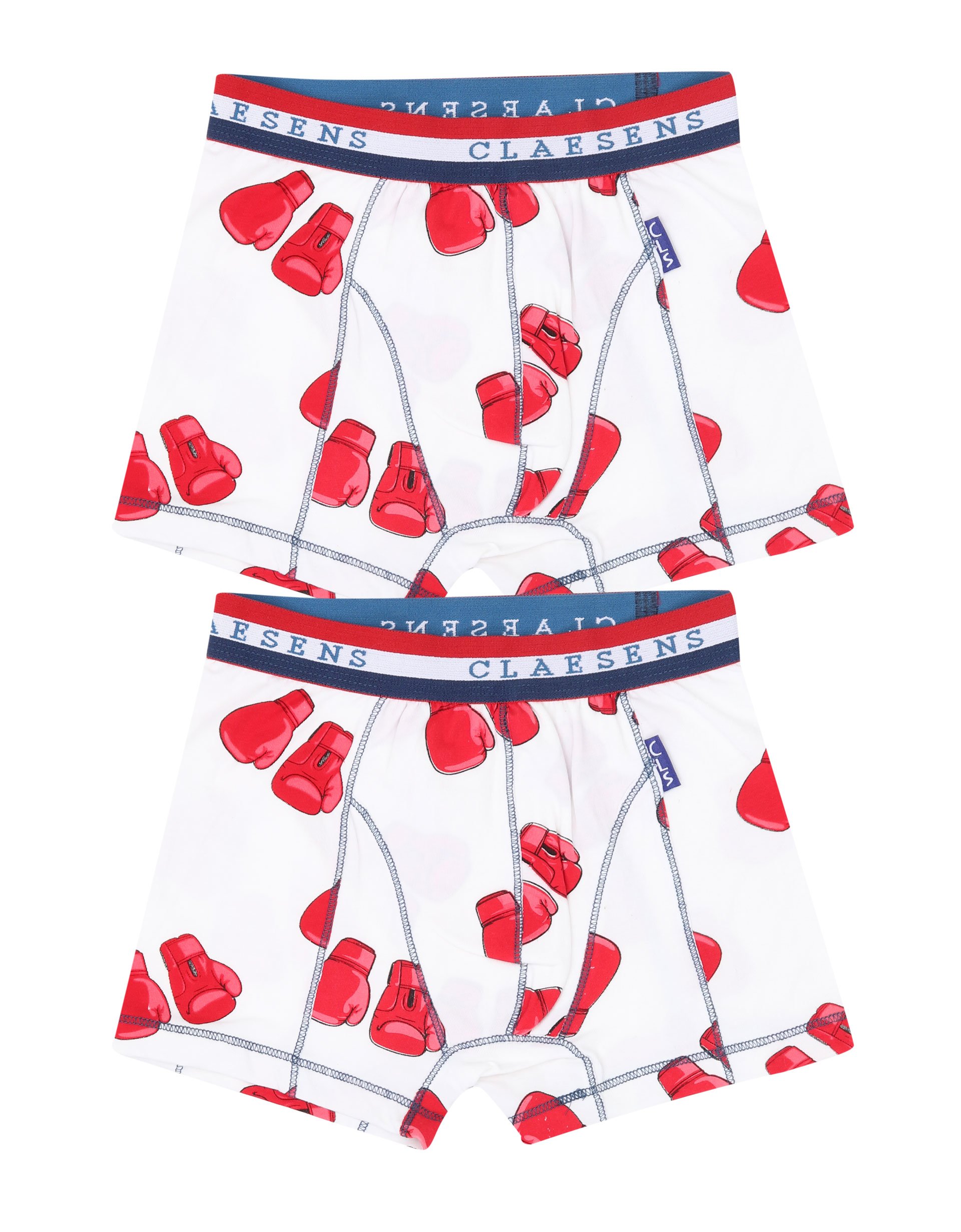The image features two pairs of men's boxer shorts meticulously laid out flat against a stark white background, creating a clean and focused advertisement-like display. Both pairs are centrally positioned with one pair placed directly on top of the other. The design prominently features a pattern of red boxing gloves scattered across a white fabric. The waistband is distinguished by a tricolor stripe pattern: a bold red stripe at the top, a white stripe in the middle bearing the brand name "Claessens" in blue text, and a blue stripe at the bottom. This branding detail is further reinforced by a small blue tag on the inside of the waistband, repeating the name "Claessens." The boxer shorts also show detailed stitching, enhancing their crafted appearance. Overall, the vivid colors of red, white, and varying shades of blue, along with the playful boxing glove motif, suggest a blend of sporty humor and high-quality design intended for a marketable product presentation.